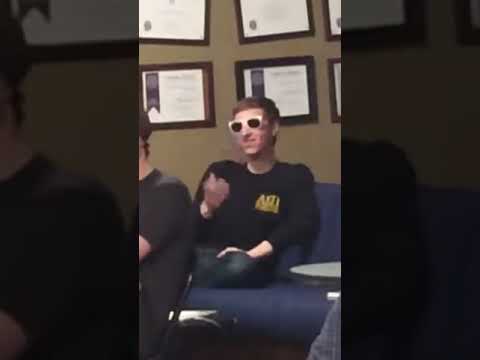In this detailed indoor scene, the image is divided into three vertical panels. The central panel, larger than the two flanking it, prominently features a man seated on a blue sofa. He sports white-rimmed sunglasses despite being indoors, has short brown hair, and wears a dark sweater adorned with yellow lettering over the left chest area. One of his hands rests on his knee while the other is held up in front of his right shoulder, potentially in a gesturing motion. Partially obscuring him from the viewer's perspective, another person is seated slightly closer to the camera; only their shoulder, upper arm, and the back of their neck are visible, as they appear to wear a dark shirt. The background reveals a brownish-tan wall decorated with two rows of three framed certificates or diplomas. The left panel is darker, showcasing only a fragment of a person - specifically their head and left shoulder - against a backdrop of the same wall. The right panel is similarly dim, presenting a portion of an individual's shoulder and arm against the wall adorned with the framed accolades. The overall ambiance suggests a setting such as a college or workplace. The notable colors include blue, tan, white, dark blue, brown, and dark brown.